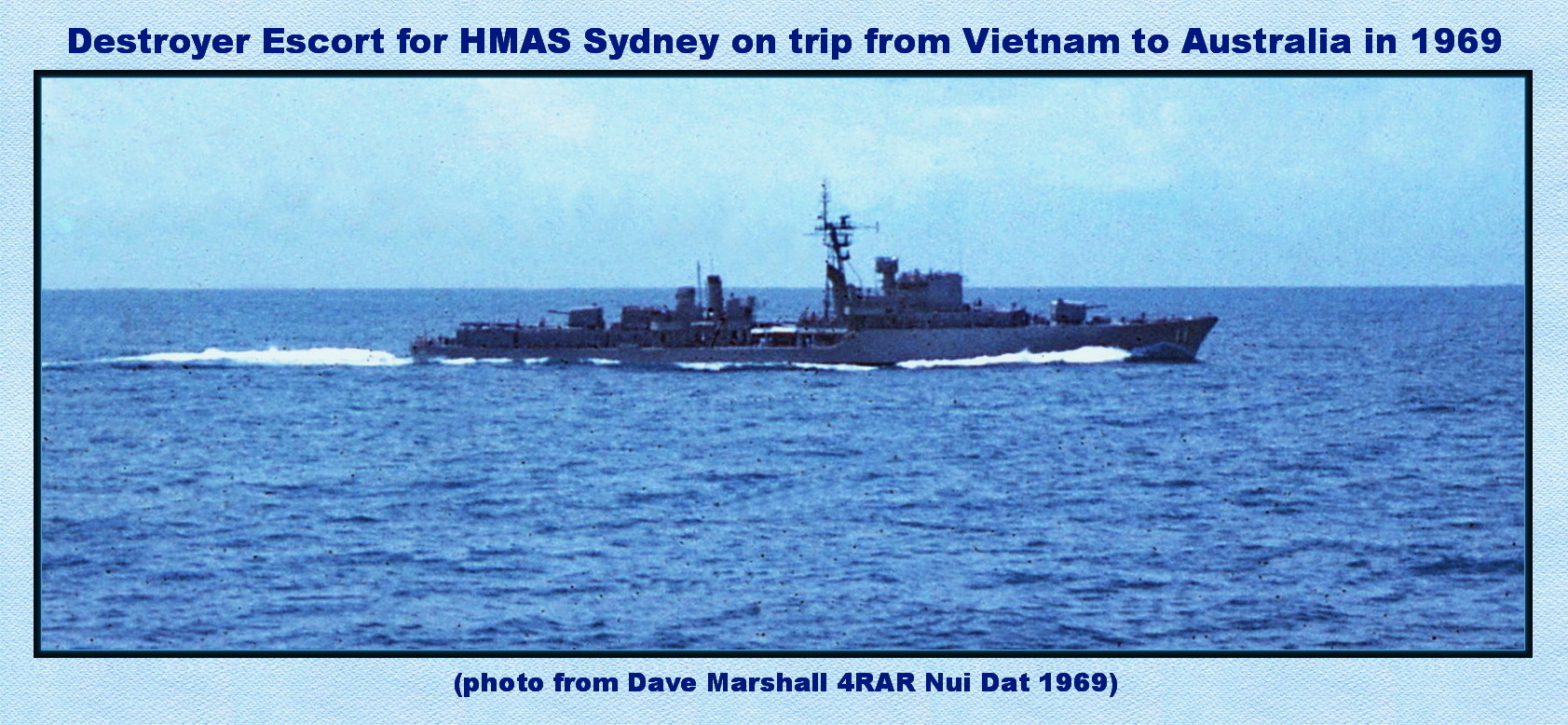This detailed image captures a large destroyer escort, identified as HMAS Sydney, on its route from Vietnam to Australia in 1969. The sky is a light, bright blue with faint clouds, providing a serene backdrop. The ocean beneath is also a vivid blue, with white waves churned up by the ship's passage visible along its sides and trailing behind it. The ship itself, appearing grey-blue and situated further back in the photograph, contrasts against the calm, expansive sea. The top of the image features a bold navy blue caption: "Destroyer Escort for HMAS Sydney on trip from Vietnam to Australia in 1969," while the bottom includes a parenthetical credit: "Photo from Dave Marshall for RAR, NUI DAT, 1969." Despite the photo's age, it remains remarkably clear, allowing for a decent amount of detail to be discerned on the ship.